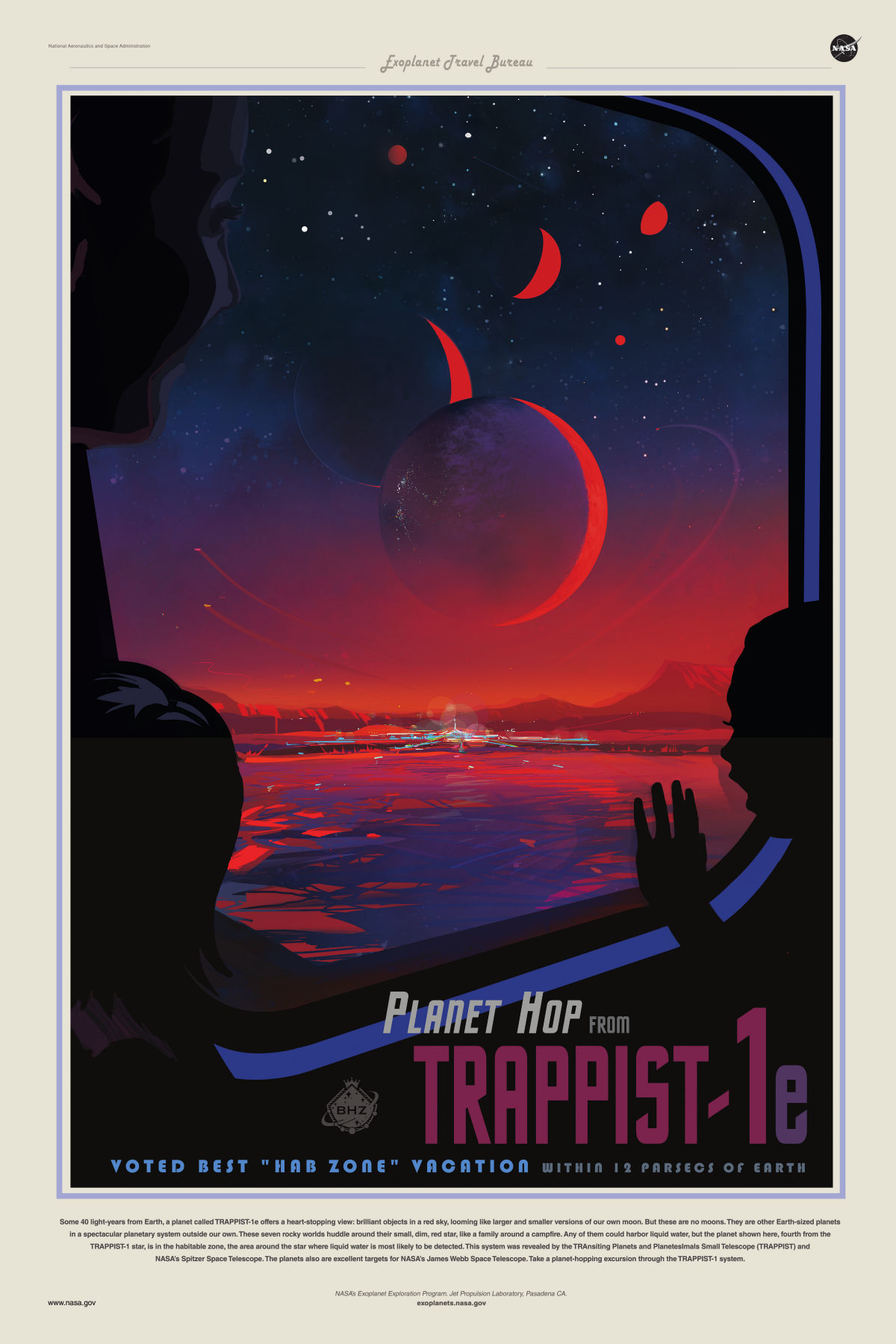This large rectangular poster, with a space vacation theme and a futuristic style, vividly depicts an adult and two children gazing out a square window of a spacecraft. They are silhouettes against a bright red-hued sky. Outside, a magnificent celestial scene unfolds with four prominent round planets and two tiny distant ones, creating an awe-inspiring view. The poster's background features a frozen lake below, with jagged red-hued mountains and a shiny building structure in the distance. White dots and red streaks traverse the night sky, adding a stellar effect. At the bottom right, the poster reads, "PLANET HOP from TRAPPIST-1-E," followed by "VOTED BEST HABZONE VACATION WITHIN 10% OF THE EARTH" in smaller letters. The thick white border at the bottom and a thinner white border around the sides frame the mesmerizing scene, while small black writing subtly adorns the bottom edge.